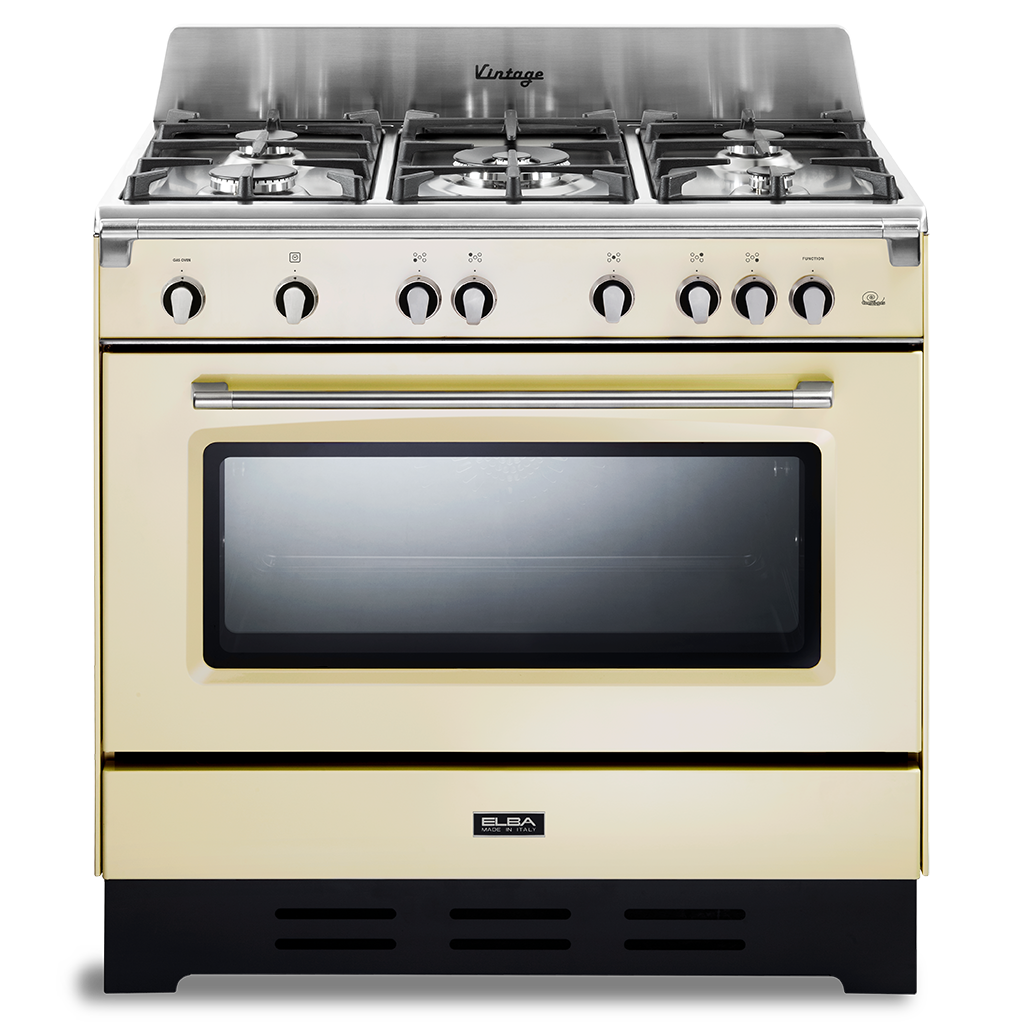This image depicts a silver metal six-burner gas stove with a mix of beige and light tan accents. Prominently marked with the word "vintage" in black print on its stainless steel backstop, the stove features three rows of two burners each on the cooktop. The front panel hosts eight knobs for controlling the burners' heat settings. Below the knobs, a silver handlebar opens to reveal an oven with a window framed in black, allowing a view into the gray interior. The bottom section includes a lower drawer for storage, and the base of the stove is black with two black feet on either side. The stove's brand, "Elba made in Italy," is subtly indicated on a small black plaque with white lettering. The background of the image is white, ensuring all details of the stove are clearly visible.